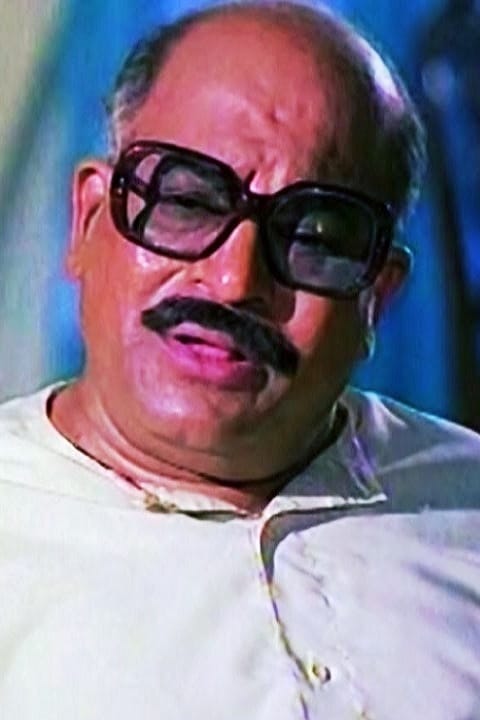The image is a color photograph in portrait orientation, capturing a man in his 50s or 60s from the top of his head to mid-chest. The man, who appears rather thickset, has a receding hairline with patches of black and gray hair on the sides of his head. He wears large, heavy-rimmed black rectangular glasses that are slightly tinted. His reddish-brown complexion is complemented by a neatly trimmed mustache. He is dressed in a light cream-colored pullover shirt with the collar slightly turned back and the top one or two buttons undone. The man’s mouth is slightly open as if speaking, and he gazes downward and slightly toward the viewer. The background is predominantly blue but blurred, making it difficult to discern the location. The photograph is stylistically representational with a focus on realism.